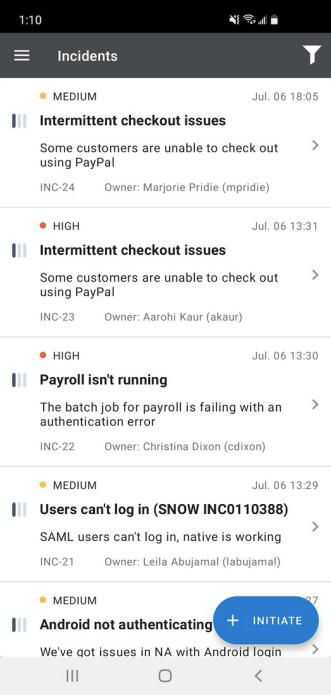The image is a vertical screenshot taken from a smartphone. At the very top, there is a black bar displaying the current time as 1:10 PM in the upper left corner, followed by various status icons on the right such as signal strength, Wi-Fi signal, and battery life. Below this is a gray navigation bar with three horizontal lines indicating more options on the upper left side, alongside the word "Incidents" in white font. On the right-hand side of the gray bar, there is another white icon.

Following this header, the content of the screen is divided into several sections, each highlighted by either an orange or red dot with corresponding labels such as "Medium" or "High". The first entry, marked with an orange dot and labeled "Medium," is timestamped July 6, 18:05. It briefly describes an issue: "Intermittent checkout issues. Some customers are unable to check out using PayPal." This issue is identified as INC 24 and owned by Marjorie Pretty, abbreviated as MPRI DIE.

The next entry features a red dot labeled "High" and timestamped July 6, 13:31. It notes another intermittent checkout problem, again with customers unable to use PayPal. This issue is listed as INC 23 and is under the care of Arolli Carrar (ACower).

The third entry, also marked with a red dot and labeled "High," addresses a payroll error: "The batch job for payroll is failing with an authentication error," including the details of its owner.

Next is another "Medium" issue indicating that "Users can't log in." It highlights that while native users can access the system, SMA users are experiencing login failures.

The last listed issue is also marked as "Medium" and relates to an unspecified authentication problem on Android.

At the bottom of the screen, there's a blue button labeled "Initiate" accompanied by various icons.

This highly detailed screenshot captures an array of system issue logs, providing insight into multiple ongoing technical problems and their respective severities and timestamps.